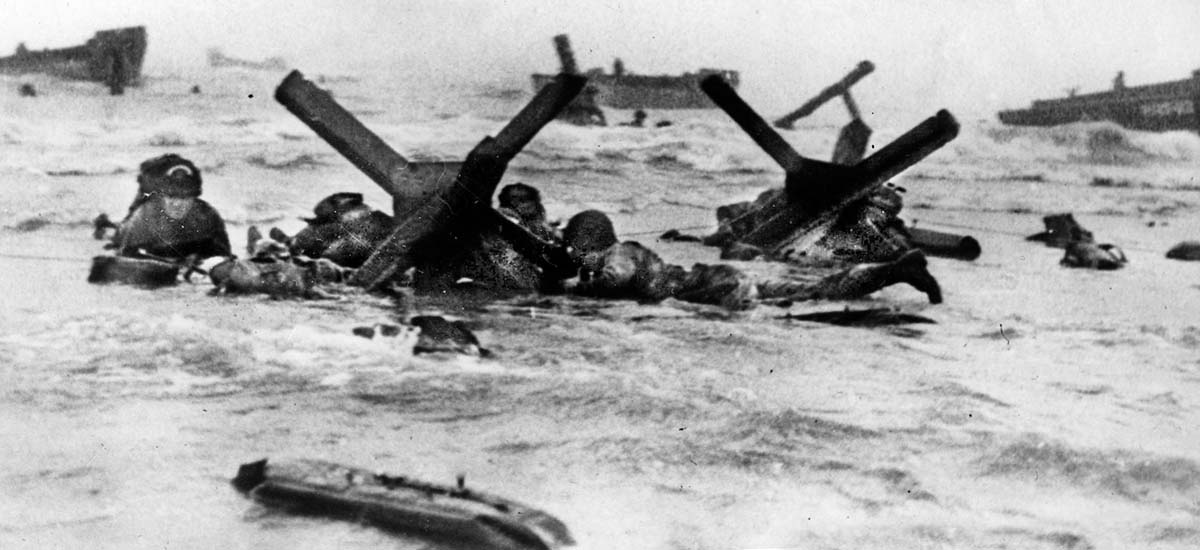In this black and white photograph from D-Day, soldiers are seen in shallow, receding water, lying behind or beneath wooden fortifications known as X-shaped crosses or metal spikes. These structures provided cover against enemy fire. The scene is chaotic, with several soldiers positioned on their bellies, appearing to cling to these barricades. The background reveals multiple boats that delivered the troops to the shore. Various pieces of wood, possibly debris or bodies, float nearby, further highlighting the aftermath of the landing. The photograph, distinctly old, captures the grim reality of this pivotal World War II moment, though the lack of color and clarity makes it difficult to ascertain all details precisely.